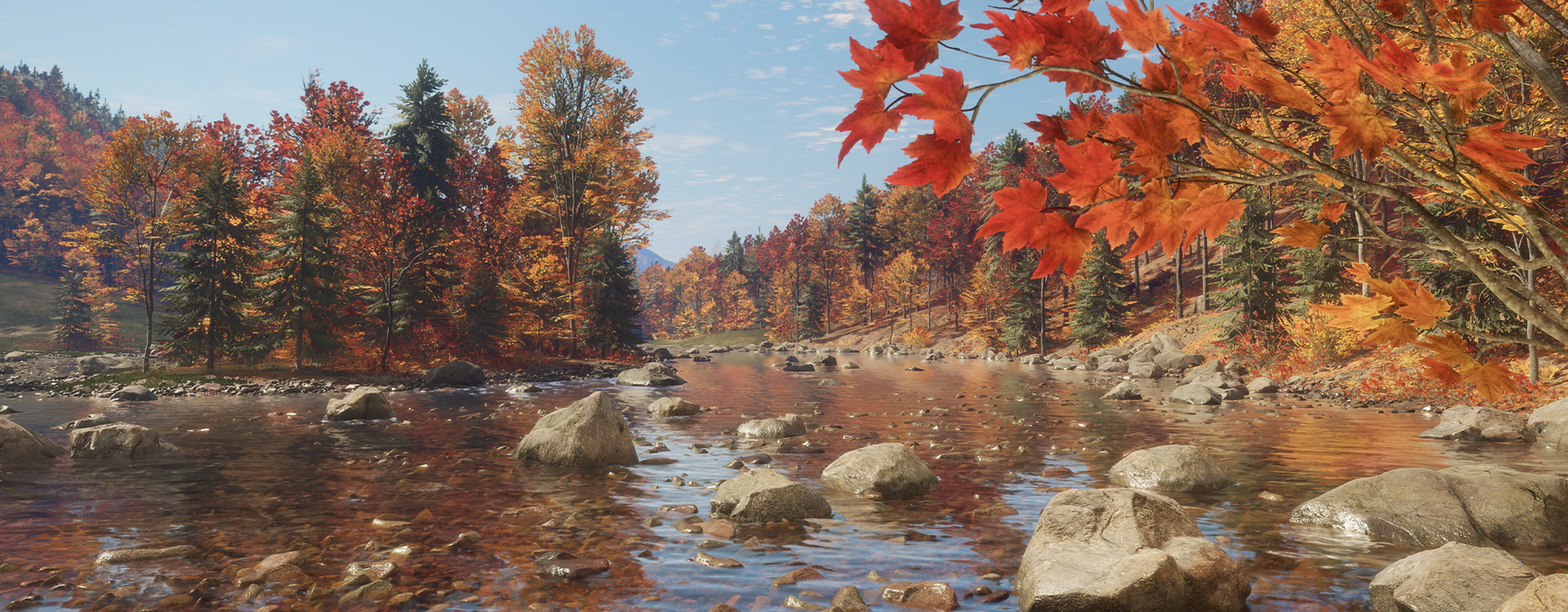The photograph captures a serene autumn scene of a shallow creek, its banks lined with an array of rocks varying in size, some protruding out of the water. The clear, calm water reflects the sky and the bordering trees. In the background, towering Douglas fir trees and other evergreens stand in contrast to the vibrant fall foliage. The leaves on the trees and ground showcase a spectacular palette of red, orange, and yellow hues, indicating the peak of the autumn season. There are patches of greenery amongst the largely autumn-colored landscape, providing a rich tapestry of seasonal transition. On the right side of the image, the ground is carpeted with fallen leaves, intensifying the autumnal feel, while the left side displays more lush, green undergrowth. The scene is framed as though the viewer is at a low vantage point, almost ground level, drawing attention to the interplay of the natural elements and the changing seasons.